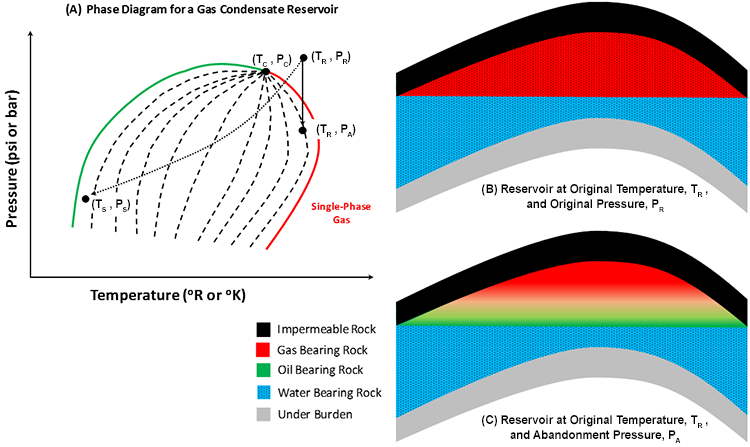This image contains a detailed composite of multiple charts and graphics related to a gas condensate reservoir study. In the top left corner, Chart A is a phase diagram for a gas condensate reservoir, illustrating the relationship between pressure (psi or bar) and temperature (degrees R or K). This chart features several curved lines, with the outer line on the left in green and the outer line on the right in red, along with four marked points using black dots.

To the right, there are two additional charts labeled B and C. Chart B is titled "Reservoir at Original Temperature and Original Pressure," while Chart C is titled "Reservoir at Original Temperature and Abandonment Pressure." These charts display stratified layers with different color codes: black for impermeable rock, red for gas-bearing rock, green for oil-bearing rock, blue for water-bearing rock, and gray for the underburden. Each chart layer is represented by a wave-like pattern, providing insights into the reservoir's composition at different pressures.

Accompanying the charts, there’s a table indicating what various colors mean for these geological layers. This comprehensive illustration supports a thorough understanding of the phase behavior and material distribution within a gas condensate reservoir at different pressure conditions.